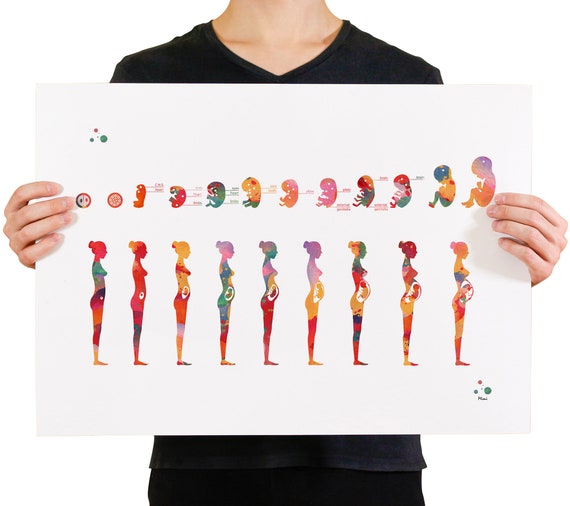The image depicts a person, potentially a woman, wearing black slacks and a black V-neck t-shirt. Their head is cropped out of the frame, revealing only their neck and hands. The individual is holding a large white piece of paper with both hands. This paper features a detailed, colorful depiction of the stages of pregnancy. At the top section of the paper, there are approximately 12 images illustrating the development of an embryo, starting from a single cell and progressing through various stages until it becomes a full-grown baby. Below this, another series of images, about 9 in total, showcases a woman at different stages of her pregnancy, with her stomach growing larger month by month. The silhouettes in these images are filled with vibrant colors such as oranges, yellows, and greens. The progression visually demonstrates the fetus’s development inside the womb, culminating in the final stage where the baby is fully developed and positioned for birth.